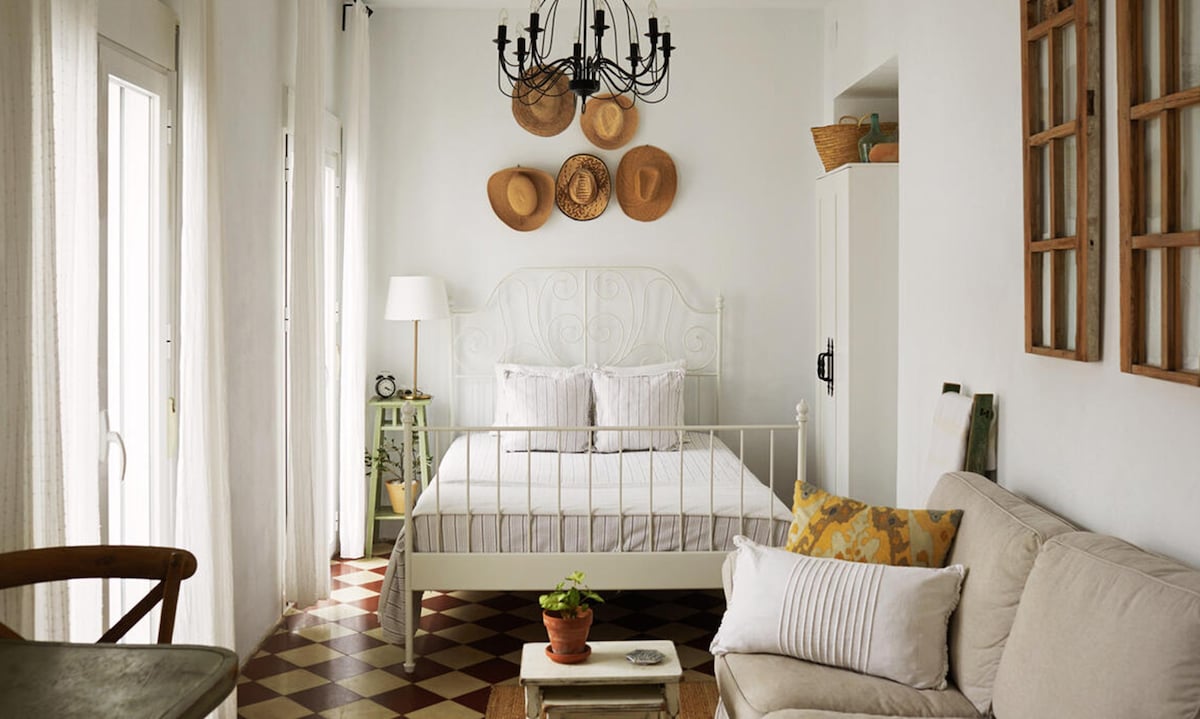A bright room with white walls features a sliding glass door on the left adorned with a pristine white curtain. On the right side of the room, against the wall, stands a beige two-cushion seat, embellished with a white pillow and a gold pillow that has a leafy design. Adjacent to the sliding door is a sturdy brown wooden table accompanied by a matching wooden chair. 

Dominating the back of the room is a white metal-framed bed, neatly made with a white mattress, white blanket, and two white pillows. Beside the bed on the left is a green stool, on top of which sits a brown lamp with a white lampshade, accompanied by a small black clock. 

Adorning the wall above the bed are five cowboy hats and an elegant black chandelier. The floor is distinctively designed with white and brown diamond-shaped tiles, adding a touch of pattern to the room. 

At the foot of the bed, a white table showcases a vibrant red pot containing a lush green plant, accompanied by a shiny silver circular object to the right of the pot.